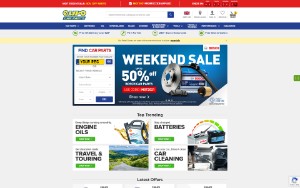This screenshot captures the homepage of an online store specializing in car parts, accessories, and essentials. Dominating the top of the page is a vibrant red bar densely packed with text. Centrally placed beneath the bar, the company’s logo is flanked by a search bar and a series of icons allowing quick access to the homepage, a favorites section, and the shopping cart.

Outlined in blue, the main navigation menu features numerous white text sections, though the specifics are illegible. Directly below the menu, four reassuring icons communicate guarantees such as fast shipping and reliable delivery.

The core of the page showcases a prominent weekend sale advert highlighting a substantial 50% discount on batteries. The advertisement, set against a blue background, prominently displays a battery pack. Adjacent to this is a section where customers can input their car’s make and model to find the appropriate battery.

Further down, a category section presents four clickable images, each representing different product categories: engine oils, batteries, travel and touring accessories, and car cleaning supplies. This comprehensive layout aims to provide a seamless shopping experience for all automotive needs.